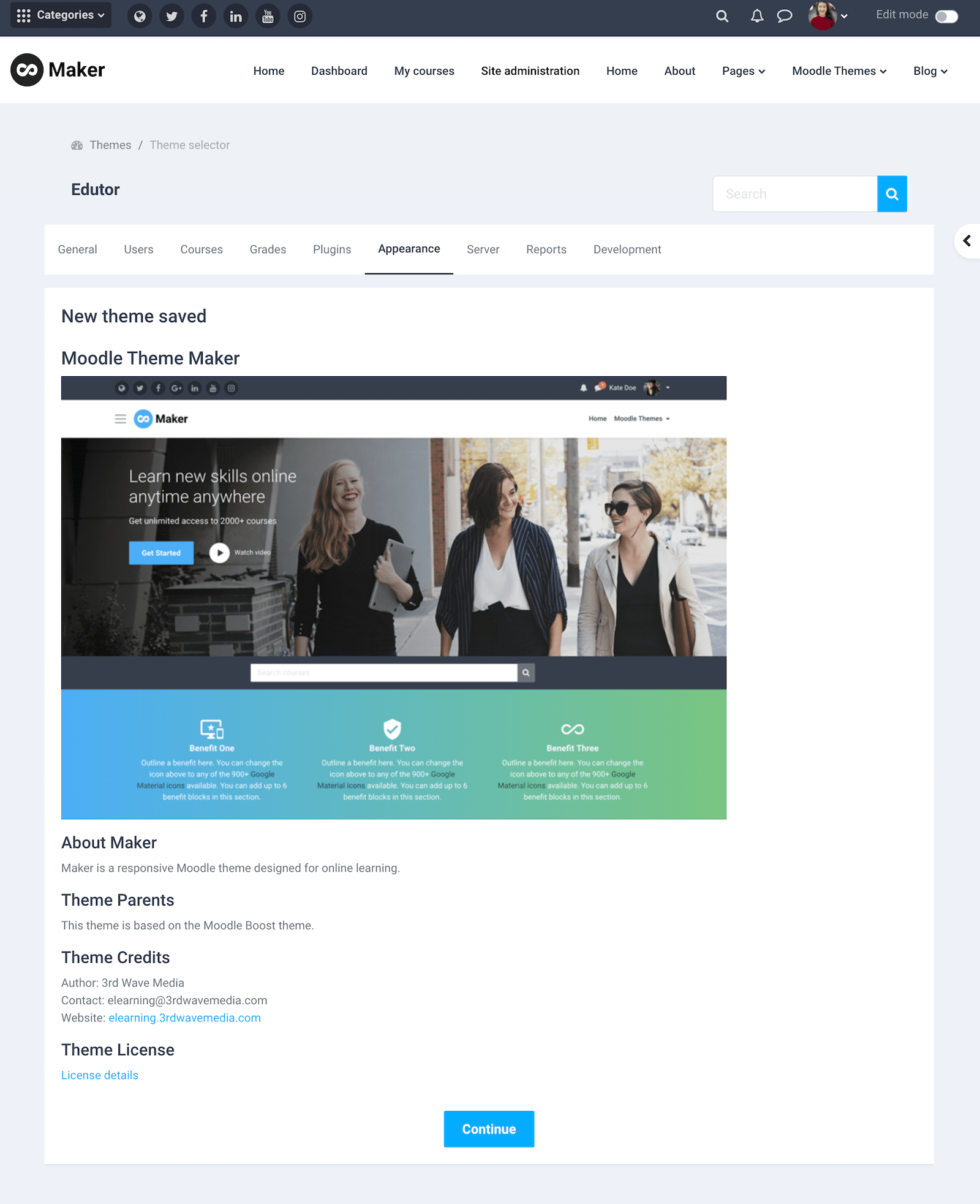The image features a screenshot of a webpage titled "Moodle Theme Maker," with an infinity symbol placed next to the word "Maker." The main message displayed is "New theme saved," indicating successful customization or creation of an educational theme on the platform. The top section of the page displays various icons, including Facebook, Twitter, and Instagram, along with a user profile logo to the right. Additionally, an 'edit mode' option is highlighted, suggesting that the user is currently editing their site.

Within the main editing window, there is a visual of a learning platform. At the top of this section, a banner says "Learn new skills online. Anytime, anywhere." Below this slogan, there's a prominent "Get Started" button meant to encourage user engagement. An image captures three women walking, smiling, and conversing in an urban environment, evoking a sense of community and collaboration.

Directly beneath the image, a search icon is displayed on a bluish-gray background, followed by three sections labeled "Benefit One," "Benefit Two," and "Benefit Three," presumably detailing the advantages of the platform. Due to the image quality, the text underneath these headings is not legible, but it likely provides further descriptions of the platform's benefits. Towards the bottom, a blue "Continue" button is visible, along with additional text that was not discernible from the screenshot.